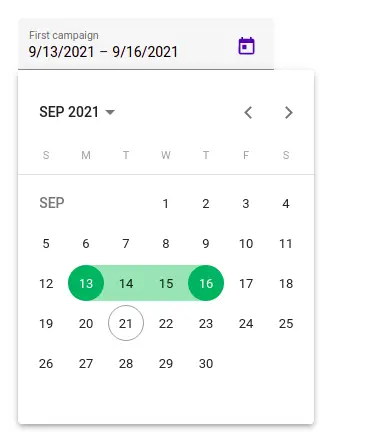The image prominently features a calendar centered in the frame, detailing a campaign titled "First Campaign." The campaign runs from September 13, 2021, to September 16, 2021, with these dates clearly denoted in black text.

At the top left corner, the title "First Campaign" is displayed, while the top right corner features a colorful calendar icon. Directly beneath, on the left side, "September 2021" indicates the current month and year. Adjacent to this, on the right, are two navigational buttons: an arrow pointing right to move to the next month, and an arrow pointing left to return to the previous month.

The calendar is structured with columns starting from Sunday on the left and ending on Saturday on the right. Notably, the current day, the 21st, is marked with a white circle outlined in gray, emphasizing that this particular Tuesday is the present day.

Selected dates for the campaign are highlighted with a green circle around the 13th (Monday) and the 16th (Thursday). Consequently, the days in between—Tuesday the 14th and Wednesday the 15th—are also shaded in green to signify the duration of the campaign.